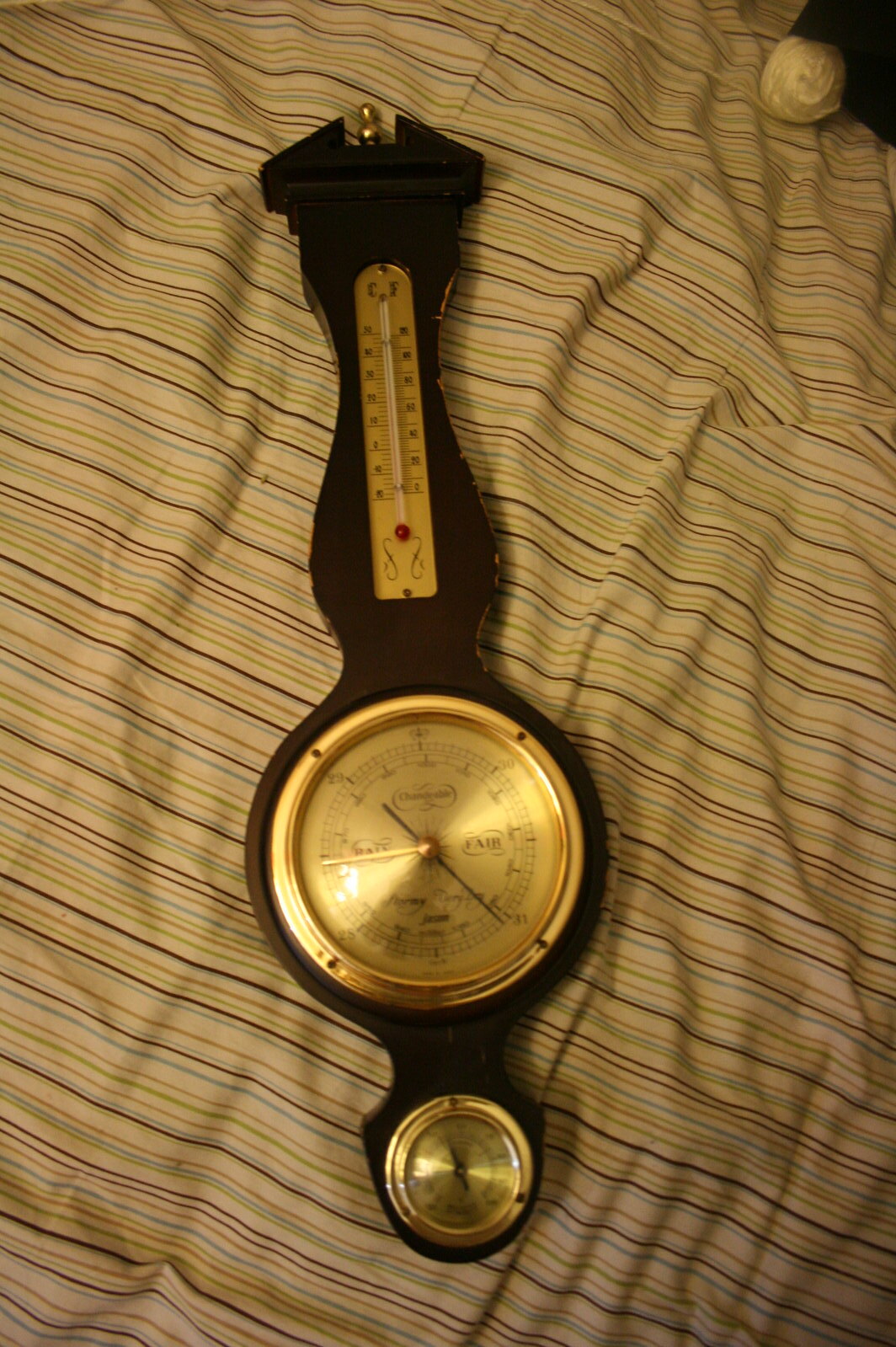The image features a detailed and vibrant blanket with multiple diagonal stripes in various colors: black, green, red, black, red, black, and blue. These stripes run diagonally from the top left to the bottom right, creating a striking pattern. 

At the top right corner of the image, there is a rubber ball that appears tied up. Centrally, the image showcases a clock face, with another clock face positioned at the bottom. Above the central clock face, there is a thermostat surrounded by a golden frame.

At the very top of the image, there is a brass metal knob attached to what seems to be a wooden handle. This handle resembles a sword when viewed from the side. At the top center, there's a tower-like glass figure, with another thermostat encased in a golden frame located in the middle.

On the left side of the image, the presumed ceiling is visible, brightly lit as if it were nighttime. The bottom of the glass figure features a red dot, and towards the center-right, the word "FAIR" is indicated, suggesting that the image involves weather measurements rather than clocks.

Dash marks encircle the elements within the image, and a smaller circle with a reflective surface can be seen at the bottom, adding complexity to the scene. Shadows on the left and right sides of the image contribute to the depth and dimensionality.